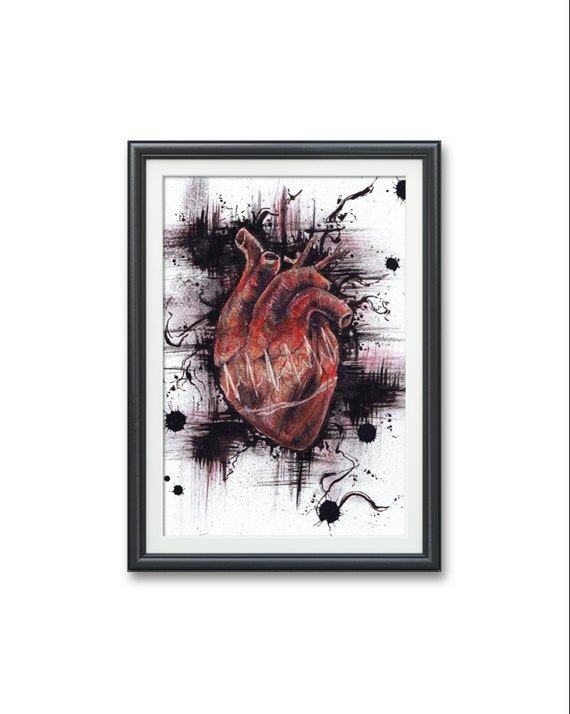The framed artwork, set against a stark white background, features a striking and somewhat disturbing depiction of a human heart, rendered with meticulous realism. The heart, in a visceral shade of red, shows detailed anatomical features, including the four ventricles and essential arteries such as the aorta, each truncated a few inches from the heart. The piece employs a mixed media approach, likely involving oil and pencil, to achieve its detailed texture and depth.

Prominently streaked across the middle of the heart in white is an EKG line, capturing the rhythmic spikes and valleys of a heartbeat, adding a clinical layer to the emotive subject. Surrounding the heart is a chaotic expanse of black paint, applied in a manner that blends cross-hatching with thick, almost inkblot-like spots, and wild, erratic paint trails, suggesting a dark, shadowy energy or turmoil emanating from the heart. The background is a turbulent mix of black and dark red, enhancing the piece's ominous and heavy atmosphere.

The entire composition is matted with a white inner border that contrasts sharply with the darkness of the painting, all encased in a simple, yet striking black frame. This piece could be interpreted as a metaphorical exploration of heartbreak or physical illness, imbued with a sense of emotional or physical trauma, making it a powerful and evocative visual experience.